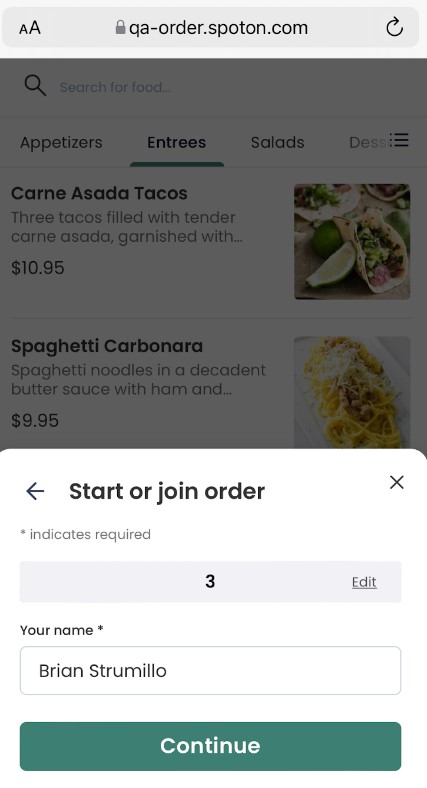The image is a screenshot from a mobile device displaying a food ordering webpage. At the top, a light gray search bar features a pair of uppercase 'A' icons on the left for adjusting font size, and a padlock icon, signifying a secure connection next to the URL "qa-order.spoton.com." A circular arrow icon is positioned to the right to refresh the page.

The upper half of the screen has an opaque gray overlay. Beneath this, a search prompt reads "Search for food" next to a magnifying glass icon. Below, menu categories such as "Appetizers," "Entrees," "Salads," and "Desserts" are listed, with "Entrees" currently highlighted. The menu displays items including "Carne Asada Tacos," described as "Three tacos filled with tender carne asada garnished with..." priced at $10.95, accompanied by a photo on the right. Another item, "Spaghetti Carbonara," also includes a description, price, and image.

A white semi-transparent box with an 'X' at the top right corner, allowing it to be closed, overlays the menu. It prompts the user to "Start or join order," with a numeral "3" indicating either the number of people or items. An option to edit this number is provided. Below, a required field labeled "Your name" with an asterisk is filled in with the name "Brian Strumillo." At the bottom, a teal bar spans the width of the screen with the word "Continue" in white, signifying the button to proceed with the order.

This comprehensive image provides a clear, step-by-step guide through the food ordering process on the platform.